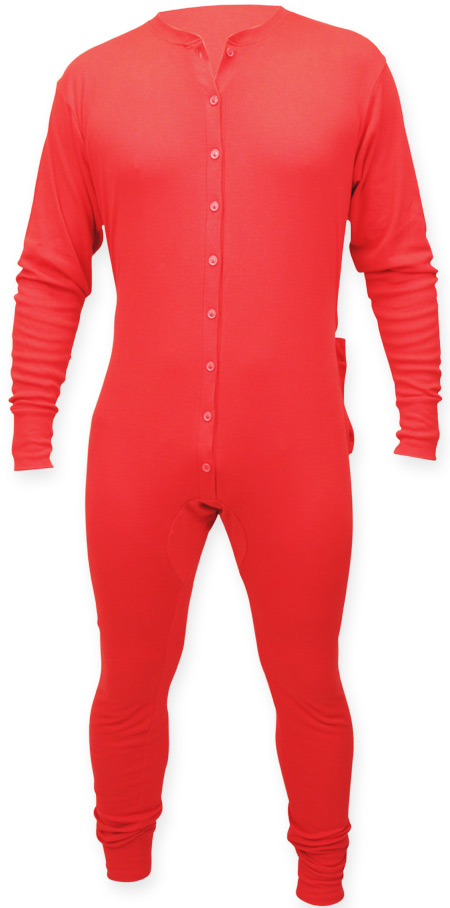This image, taken in a portrait orientation, depicts a vibrant red adult onesie pajama set, reminiscent of classic long johns. The garment is a single-piece outfit featuring long sleeves and full-length pants that taper tightly at the ankles, adorned with ruffles just above. The fabric shows some natural wrinkles, particularly along the arms, which are positioned to the sides. The front of the onesie has a series of buttons starting from the simple, rounded collar and extending down to the crotch. Notably, the top button is unfastened. On the right hip, there's a noticeable protrusion, likely indicating a rear flap with a button, typical for convenient restroom use. This classic winter wear stands out against a stark white background, highlighting its bright red color.